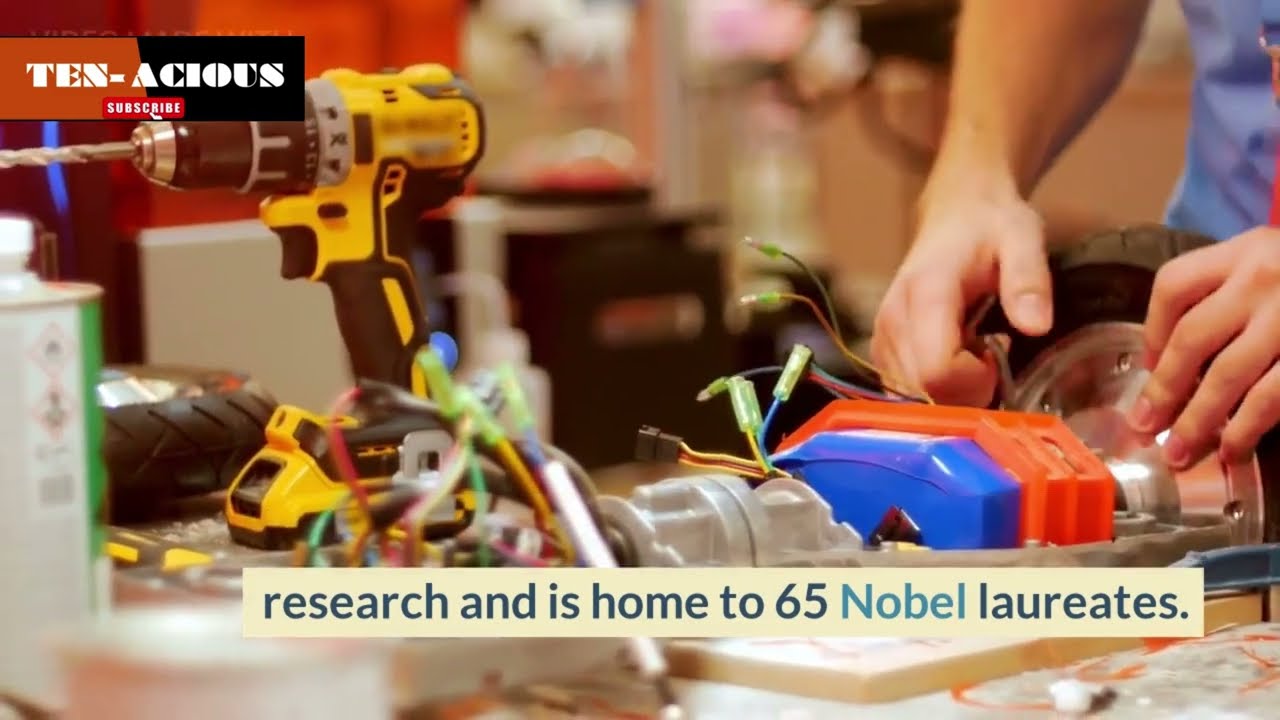The photograph captures a detailed scene of a workbench in what appears to be a bustling workshop or engineering lab. At the center of the image, various hands are engaged with tools and materials, suggesting focused activity on an electrical engineering project. A blue-shirted individual, partially visible only by his arms and hands, is working on a shiny black tire with a silver rim, surrounded by a collection of colorful boxes—orange, blue, and steel—filled with wires. Nearby, a yellow and black cordless power drill is prominently placed on the table.

The upper left corner of the image features the text "10-ACIOUS" along with the word "subscribe," hinting at a DIY or instructional context. The background is blurred but reveals other machines, adding to the workshop ambiance. At the bottom of the image, inside a tan rectangle, the text reads, "research and is home to 65 Nobel laureates," emphasizing a prestigious research environment. Additionally, a container of paint thinner is visible on the left side, further indicating the diverse projects taking place in this inventive space.